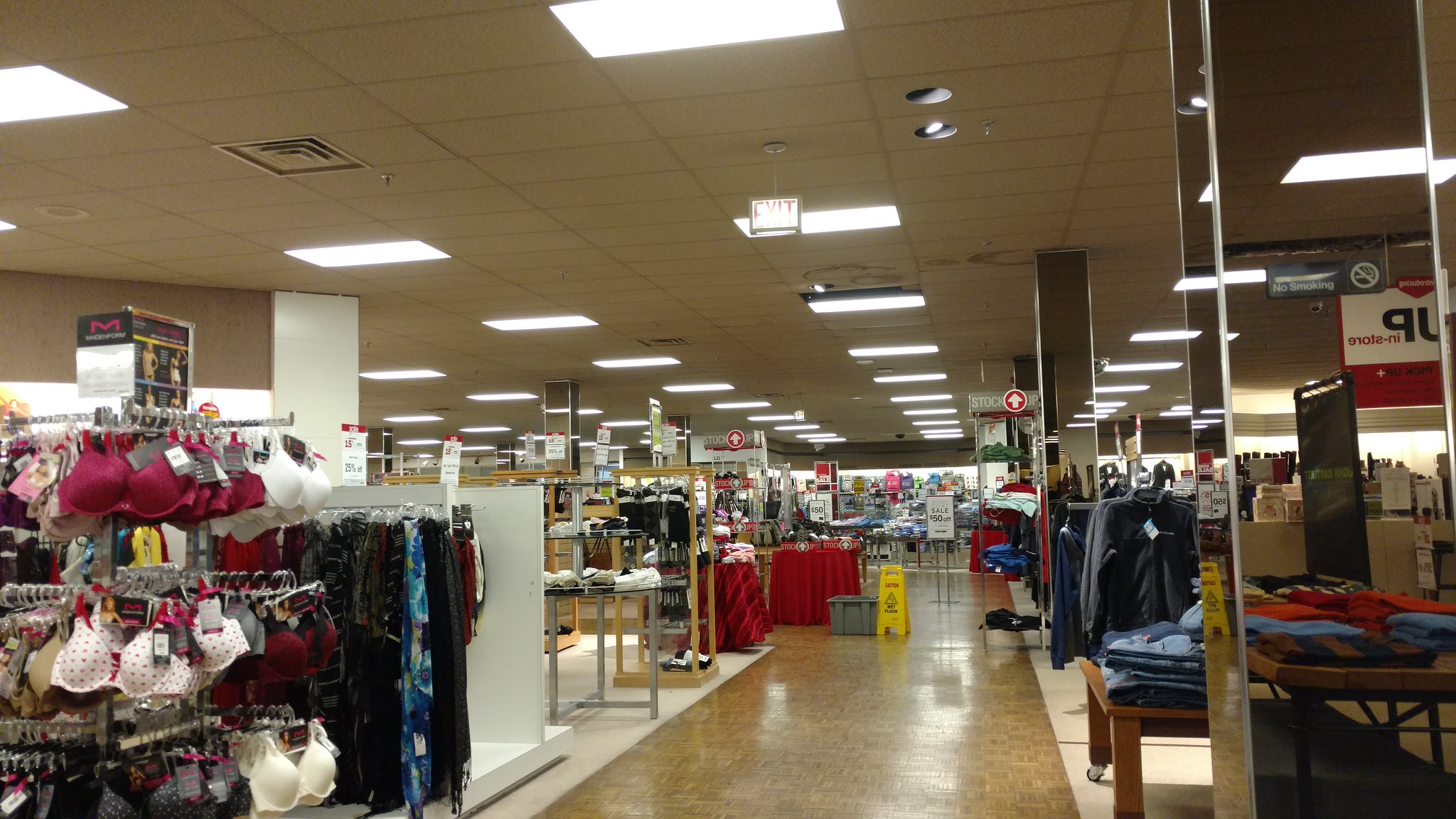This photo captures the interior of a bustling shopping center, showcasing a brown aisle that runs centrally through the scene. On either side of the aisle sit various clothing sections, each curated with a distinct selection of garments. To the left, a rack prominently displays an assortment of bras, including ones in burgundy and another with a white and burgundy polka dot pattern. Alongside the bras, a shelf holds an array of robes and pajamas, neatly hung for browsing customers. Beyond these, round tables cluttered with various items and a wooden shelf add to the diverse shopping options.

On the right, the mirrored poles lining the aisle create an illusion of expanded space, reflecting the bustling activity within the store. A cautionary wet floor sign stands ahead, signaling for careful treading. In the center of the aisle, incongruously, a gray tote has been left out. Flanking the tote, two tables draped with red cloths add a pop of vibrant color to the scene. This detailed snapshot encapsulates the varied offerings and meticulous organization within the shopping center, highlighting both the practicality and aesthetics of the retail environment.